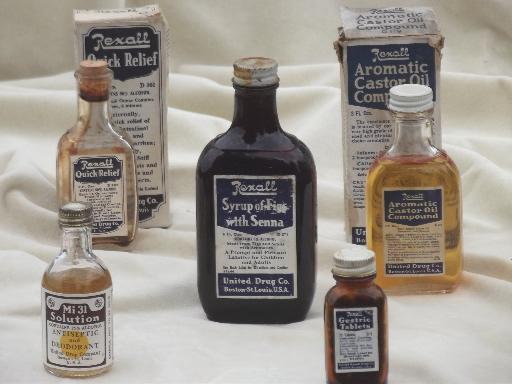The image depicts a collection of five antique medicine or antiseptic bottles displayed on a white cloth, with a white background. The largest bottle, situated in the center, is a brown glass bottle labeled "Rexall Syrup of Figs with Senna," produced by United Drug Co. in St. Louis, USA. To its right, there's a clear glass bottle filled with a yellowish liquid, labeled "Aromatic Castor Oil Compound." Below these two bottles, a smaller brown glass bottle is labeled "Gentria Tablets." To the left of the central bottle, there is another clear glass bottle labeled "Rexall Quick Relief," and to its left, another bottle marked "MI 31 Solution," which serves as an antiseptic and deodorant. Behind the bottles, there are two boxes corresponding to the Quick Relief and Aromatic Castor Oil Compound bottles. Each bottle still retains its original label and contents, showcasing a glimpse into historical medicinal practices.